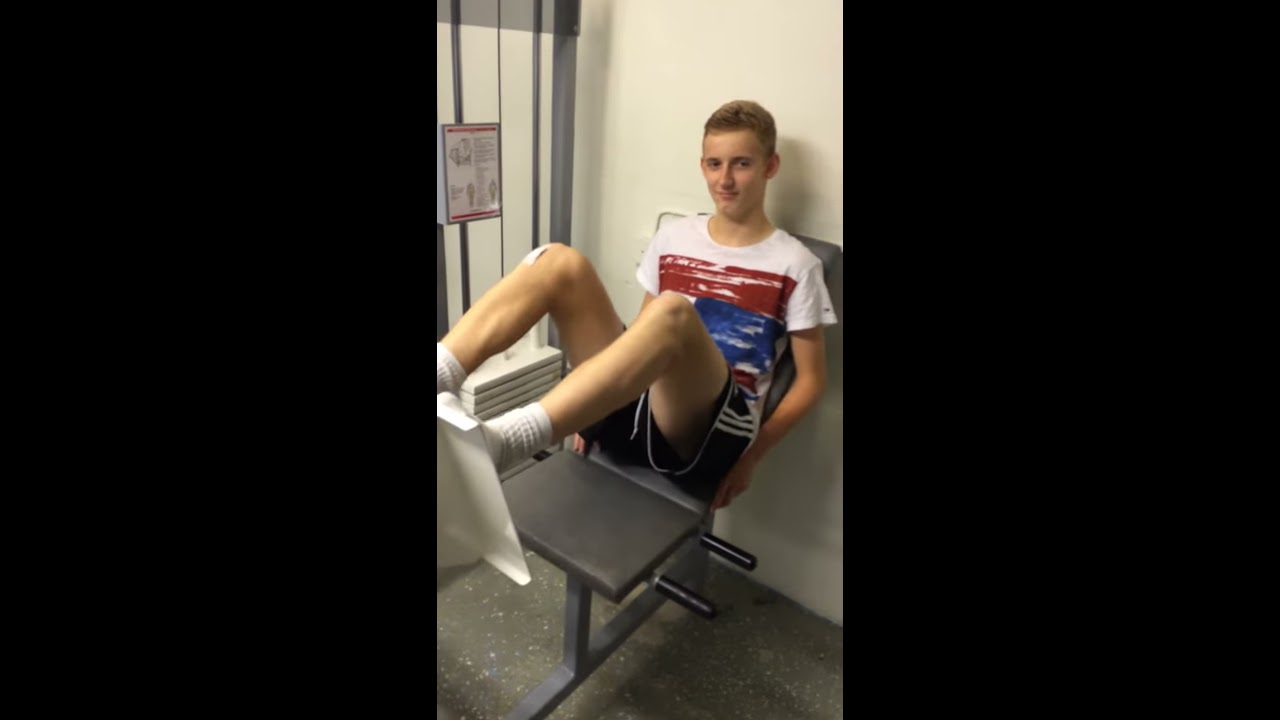A photograph captures a young man, likely in his late teens, sitting on a leg press machine in a gym. He is resting with his knees bent, as the press is currently in a fully retracted position, and his feet are propped up on a stanchion in front of him. The young man, who has light brown, short-cut hair and a handsome face with a slight closed-mouth smile, is dressed in a white t-shirt featuring a blue and red design across the chest, and black baggy shorts with white stripes down the sides. He is also wearing white socks. The gym environment includes a gray speckled floor and a white wall behind him, alongside another exercise machine with visible weights and a sign bordered in red detailing its usage. An obscured sign is also partially visible on the wall beside him.